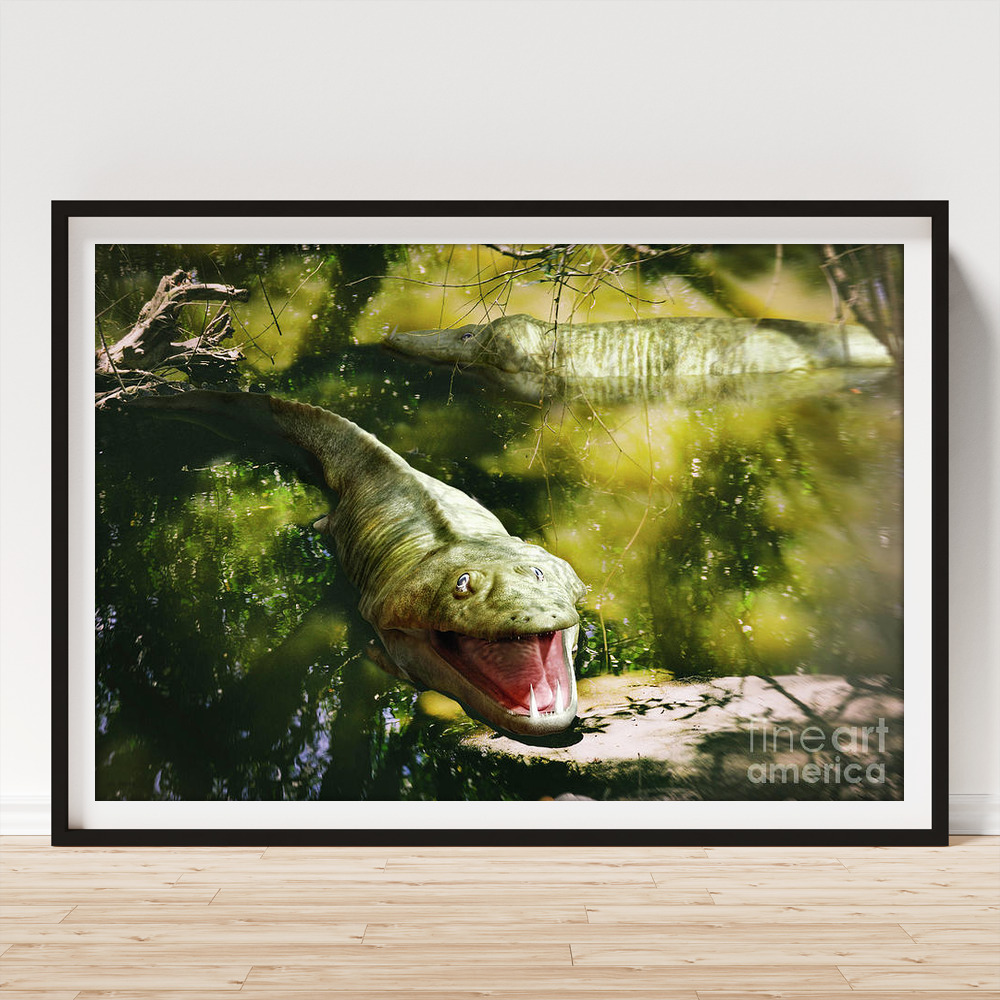The photograph captures a room with bright white walls and a light tan wooden floor, featuring a prominently displayed piece of art in a black frame. The image within the frame, credited to Fine Art America, depicts a swamp scene dominated by shades of green. Central to the artwork is a menacing, reptilian creature resembling a crocodile or alligator, yet with characteristics more akin to a snake or fish, namely lacking limbs and extending into a tail. This primary creature emerges from the swampy water, poised as if ready to strike with its open mouth showcasing sharp fangs. In the backdrop, a second, somewhat blurred, reptile is visible, leisurely swimming amidst the swamp's murky depths. The detailed artwork, bordered by a white mat within the black frame, captures the eerie stillness and predatory tension of these green-hued creatures in their habitat, complemented by reflections of tree leaves overlaying the water and a log and rock accentuating the scene's natural atmosphere.